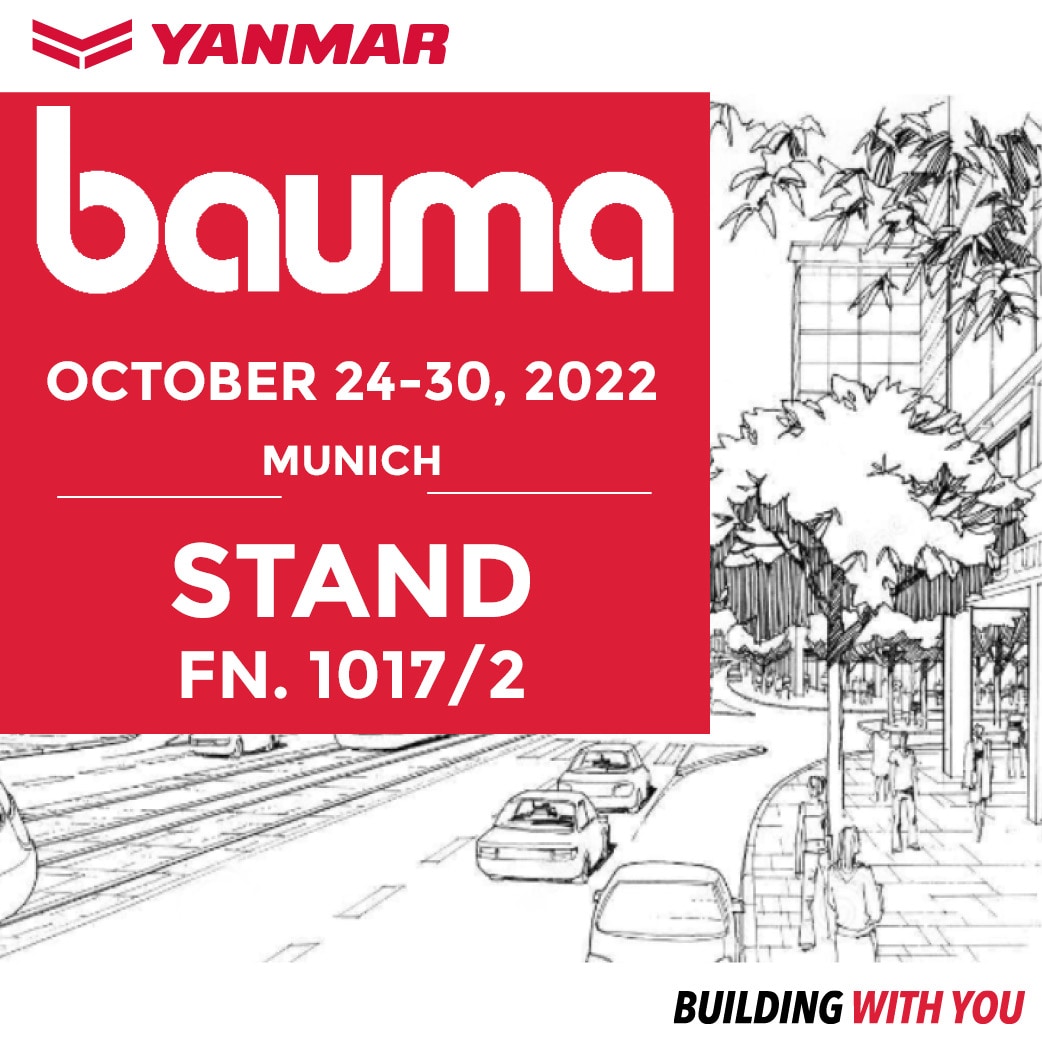This image is a detailed advertisement by Yanmar Corporation for the Bauma event, taking place in Munich from October 24th to 30th, 2022. The advertisement prominently features the word "Yanmar" in bold red uppercase letters at the top, accompanied by a logo with two V-shaped designs. Beneath this, a large red box contains white text that reads "Bauma," followed by the event dates, "October 24-30, 2022," the location, "Munich," and "Stand FN.1017-2." The background of the advertisement is a precise black-and-white sketch depicting a bustling city street. The scene includes several cars on the road, train tracks, and pedestrians walking along a sidewalk lined with trees and ornamental bushes. Impressive buildings stand tall in the backdrop, contributing to a clean and crisp urban setting. The phrase "Building with You" is displayed at the bottom right, with "building" in black text and "with you" in red text.